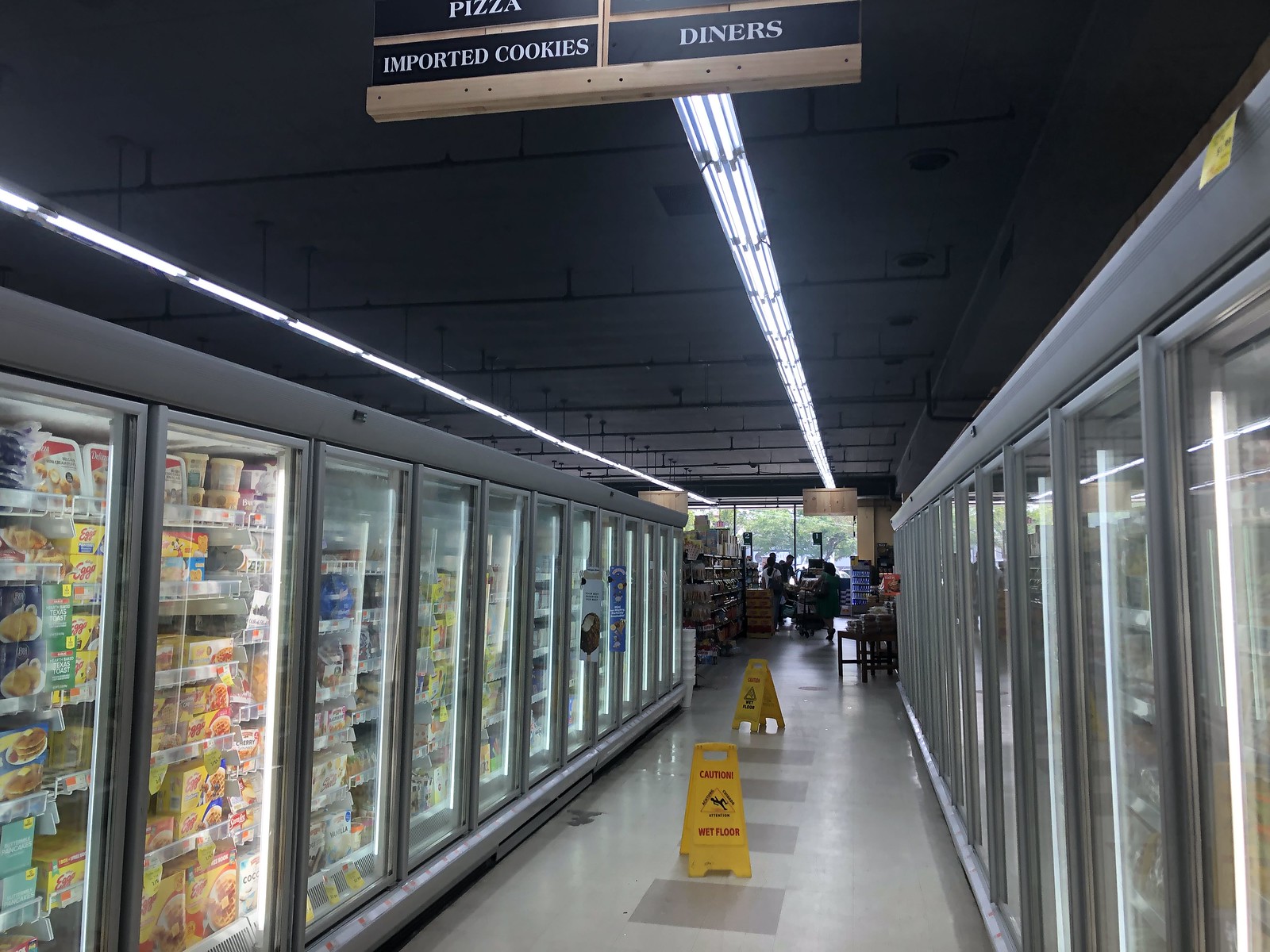The image depicts a grocery store aisle, specifically the frozen food section, characterized by floor-to-ceiling glass display cases on both sides. The aisles themselves have a mostly white floor with gray square patterns. Two yellow A-frame wet floor signs are prominently positioned in the center of the aisle. Overhead, rows of fluorescent lights illuminate the scene, and a hanging sign indicates sections for "pizza," "imported cookies," and "dinners." In the background, checkout lanes are visible along with large front windows through which trees can be seen. The photograph is wider than it is tall, and although the people in line at the checkout are present, they are not the focus and are somewhat obscured.